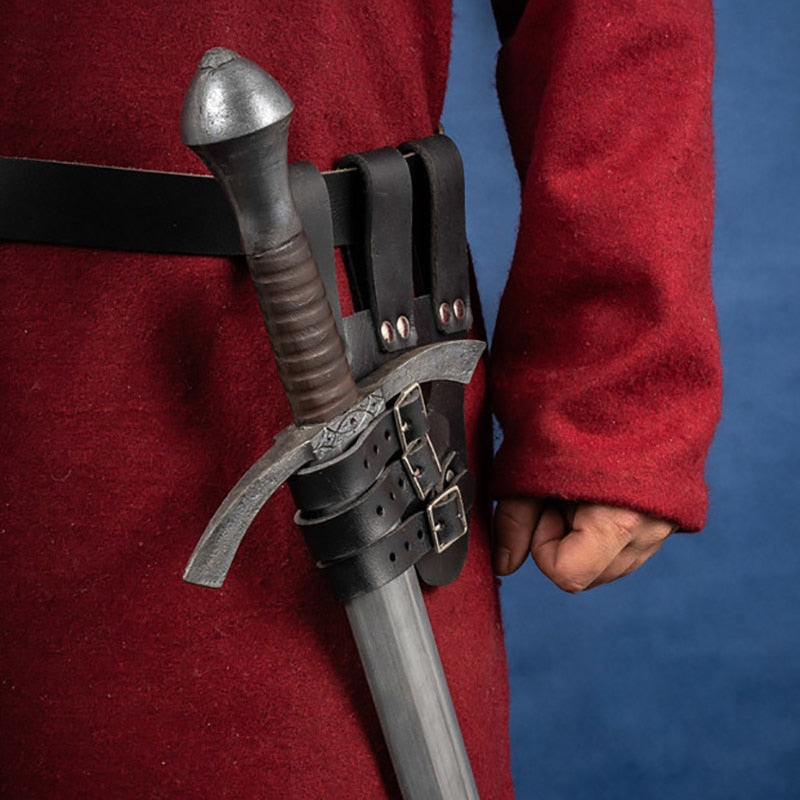The image captures the left side of a person clad in a red woolen coat, visible from just below the chest to about the thigh. The focal point is an old-fashioned silver sword sheathed in a scabbard, which is secured to a black leather belt around the person's waist by three straps. The intricately carved brown handle of the sword features hand-protecting metal elements and a knob at the top. The person's arm, positioned to the left of the image, is relaxed with fingers hanging or closed in a fist. The background is a solid blue, contrasting strikingly with the red of the coat and the metallic shine of the sword.